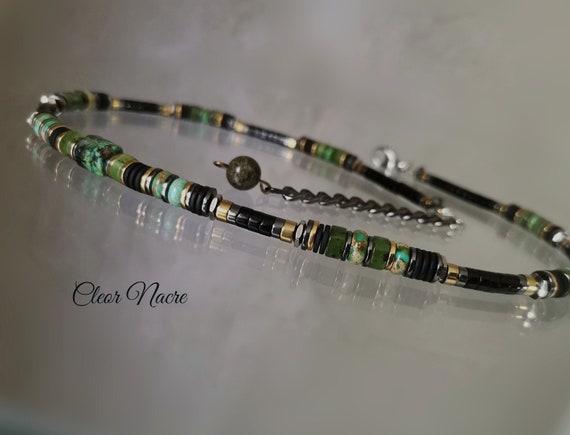The image depicts a slender, beaded necklace lying unclasped on a reflective, glass-like surface, allowing for a clear reflection underneath. The necklace, composed primarily of flat, round beads and a few square ones, features a diverse color palette including emerald, jade, teal, black, white, silver, and gold. It has a silver clasp attached to a small chain that ends in a round silver ball. In the lower left corner, there is an inscription in cursive black font that appears to say "clear NACRE," although the exact wording is difficult to decipher.